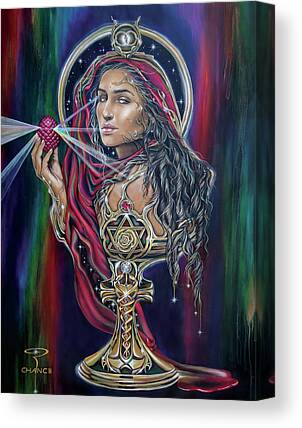This detailed painting features a mysterious, gypsy-like woman adorned in a red robe with the hood pulled up over her long, curly hair, which appears ash brown to black. Her intense, enigmatic expression suggests she holds a secret or the key to the future. She cradles an object resembling a pine cone or acorn, colored maroon or pink, emitting prisms of light or beams shooting outwards. A striking blue, nearly ethereal halo, encircles her head, adding an aura of mysticism.

The background of the painting is a dreamlike array of rainbow hues, blending and streaking together vertically. From the left-hand corner, the colors transition from red, blue, green, and dark green, shifting to bright blue at the center, then purple, and repeating again. The bottom left corner prominently displays the word "Chance" in gold, followed by a symbol of a gold swirl with a line descending from it. In contrast, the bottom right corner is solid black with drips of green and waxy red descending into it, further enhancing the painting’s surreal atmosphere.

Her attire includes Celtic-inspired jewelry, featuring what appears to be a pentagram and other intricate designs on a chalice in front of her. The portrait focuses on her from the chest up, directing attention primarily to her face and the object in her hands. The painting’s rectangular, portrait-oriented frame encapsulates this captivating blend of vivid colors, mystic symbolism, and the profound, knowing gaze of the woman.